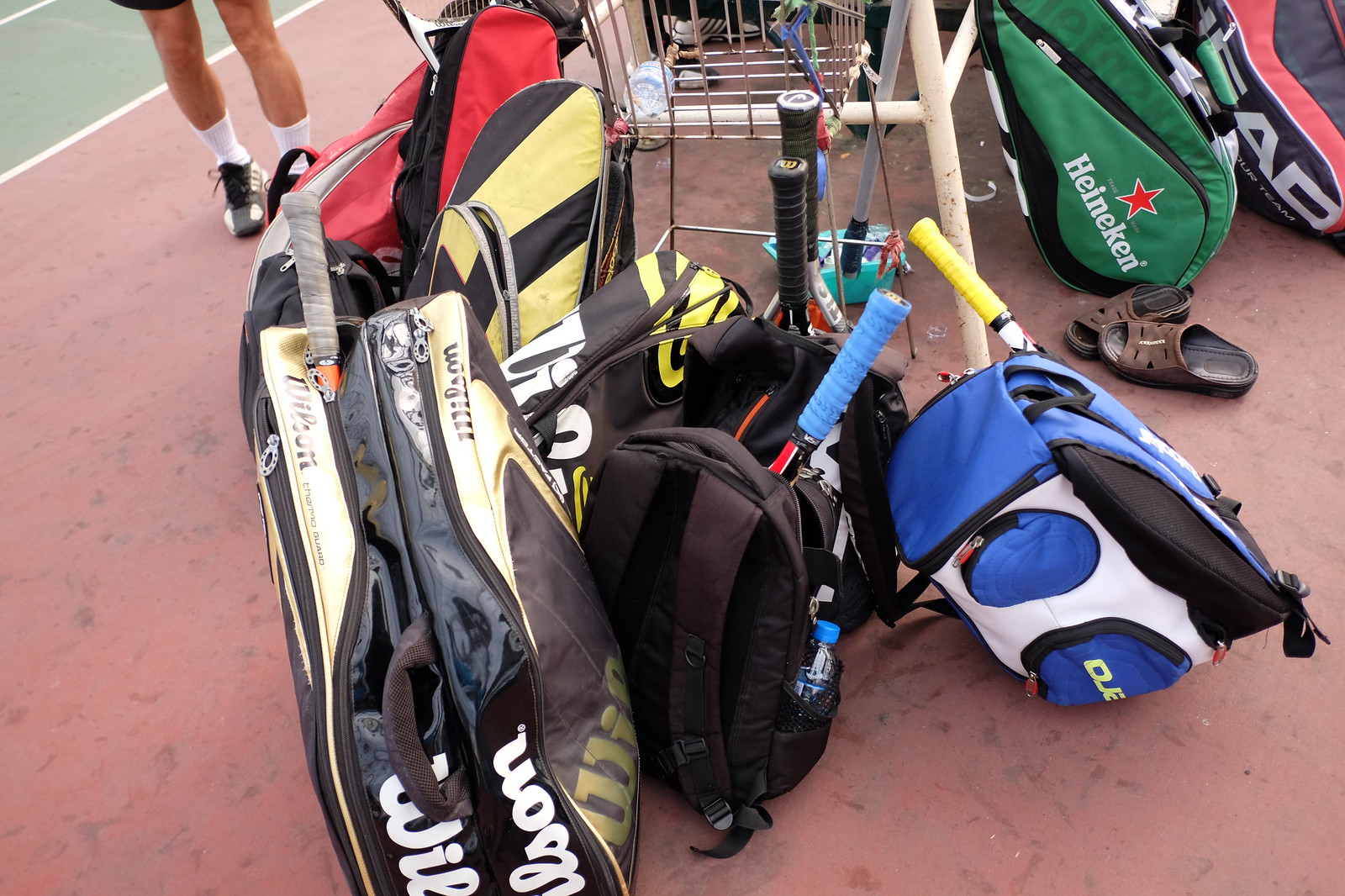In this photograph, a rectangular image captures a scene on a tennis court brimming with the assorted equipment of a tennis team. The background reveals the distinctive red surface common to tennis courts, featuring a small diagonal patch of green with white lines in the upper left corner, indicating the edge of an actual court. Prominently in the foreground, various sporting bags are scattered across the ground. These include several backpacks and duffel bags in diverse colors—black, blue and white, green with a Heineken logo, and a red and yellow striped bag. The bags are packed with tennis rackets whose handles protrude, such as one from Wilson, although the full images of the rackets are not visible. Among the equipment, there's a basket typically used for carrying tennis balls during practice sessions. Additionally, there are water bottles and sports backpacks with multiple pockets suggestive of space for shoes and other accessories. A pair of legs clad in calf-high socks and athletic shoes can be seen from the knee down, indicating the presence of a player standing nearby. Adjacent to the equipment, a pair of slides implies that someone has changed into tennis shoes. The scene suggests either a preparation for a match or a tennis lesson about to commence.